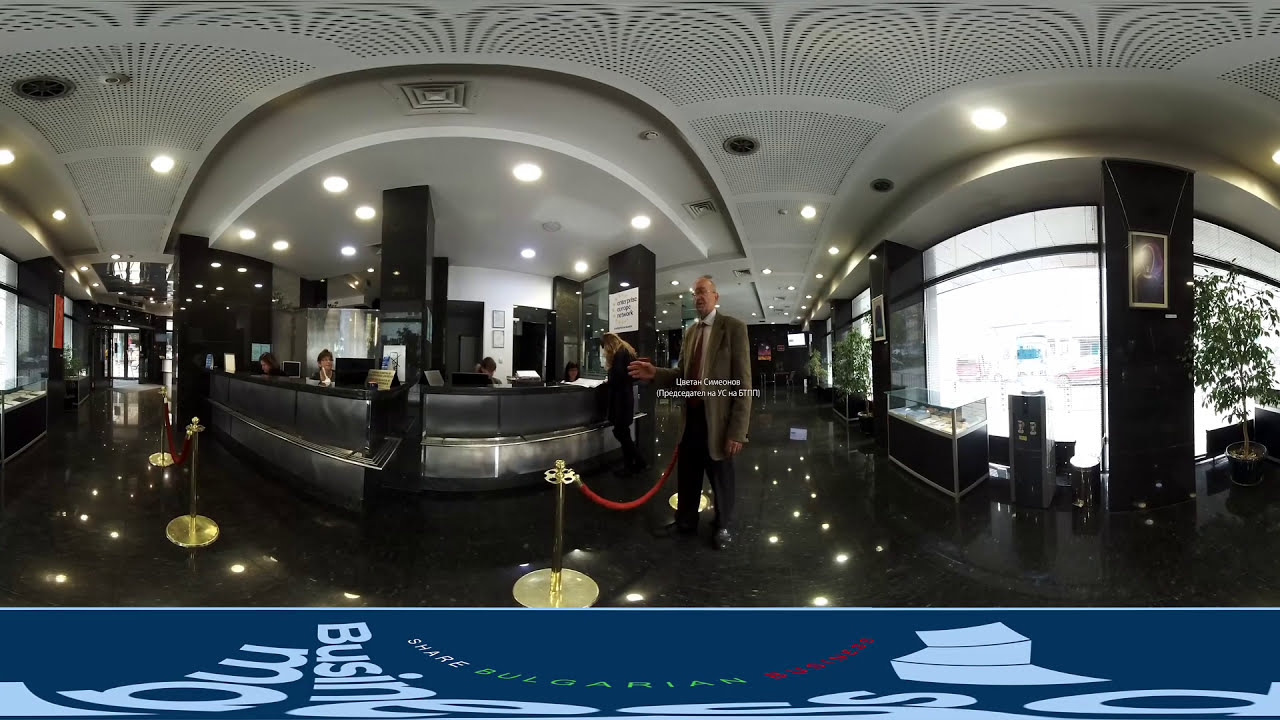The image depicts what appears to be an elaborately designed hotel lobby, likely intended to project an upscale and refined ambiance. The scene features a spacious area with a mixture of distinctive elements that create a sense of opulence and order. On the left side, a hallway extends into the distance, ending in a couple of doors that could serve as an entrance. Centrally located is a semicircular front desk, surrounded by red velvet ropes supported by gold stanchions, creating a controlled access area. To the right of the front desk stands an elderly man in a suit with a red tie, facing the viewers with his right hand extended forward as if interacting with someone or something. Behind him, another hallway recedes into the distance, and along the right side of the image, large glass walls allow in ample daylight, illuminating several green plants.

The lobby features a black or dark marble tile floor, and its ceiling is a striking white adorned with ornate designs and embedded lights. Additional architectural details include black beams and the presence of paintings or pictures on the walls. The right wall and reception area are curved, escalating the sense of grandeur. The entire scene is augmented by a dark blue border at the bottom of the image, featuring distorted text that appears digitally placed and nearly illegible but one part seems to include the word "business."